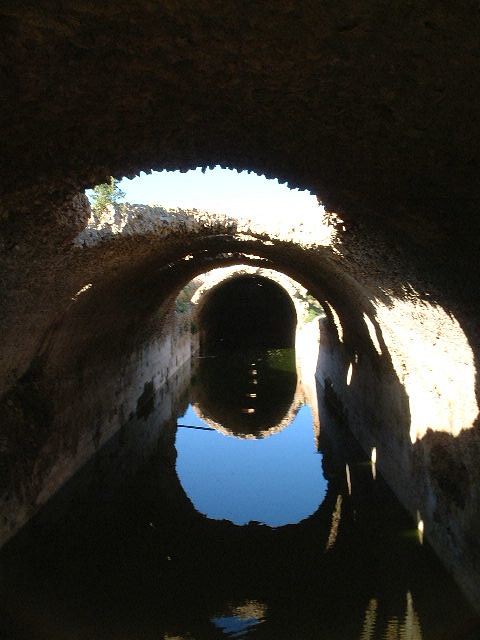The image appears to depict the view from within a tunnel or narrow passageway, possibly resembling a train tunnel. The upper section of the image is dominated by darkness, with a small strip of white below it, indicating the ceiling or arch of the tunnel. The archway itself is curved, featuring a brown hue on its upper part and beige underneath. At the center of this archway, there is a black oval shape suggesting the opening of another tunnel ahead. Below this is a blue area that resembles water, contributing to the reflection and play of light in the image. The bottom part of the image is shrouded in darkness. Additionally, there is a conspicuous area of yellow light on the right-hand side and several smaller patches of yellow light scattered around the tunnel. In the upper left corner, there are visible plants which add an element of natural surroundings to the image. The overall scene might also be interpreted as viewing upward from a cave or a hole, with an opening letting in sunlight and exposing a rugged exterior. The image combines elements of light, water, and architectural features creating a complex and somewhat ambiguous visual.